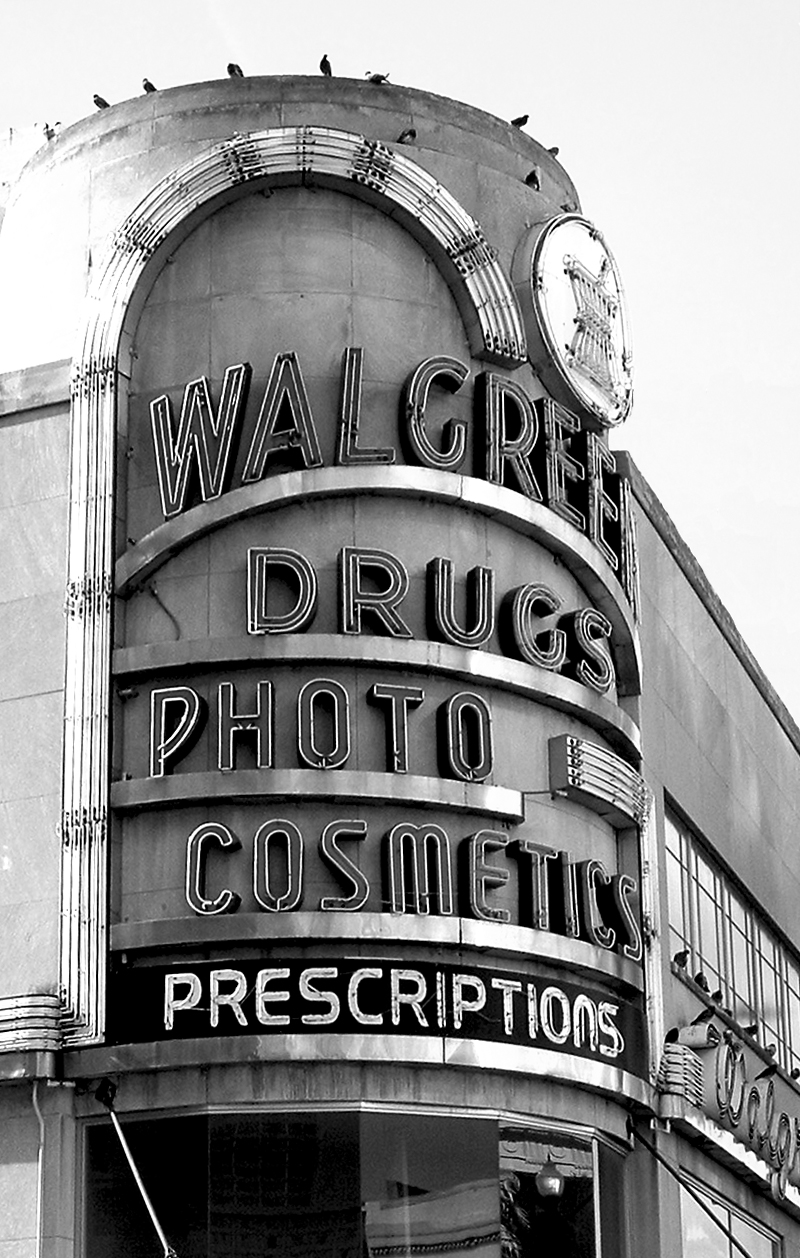A nostalgic black and white photograph captures the exterior of an old Walgreens store, likely from the 1940s based on the architectural design. The building's corner features a prominent cylindrical structure adorned with a curved, candy cane-shaped neon light that gracefully arcs to the left. Brilliant neon signs vividly illuminate the words "Walgreens," "Drugs," "Photo," "Cosmetics," and "Prescriptions," each phrase supported by its own sleek, silver beam. Approximately a dozen birds perch atop the cylindrical structure, adding a touch of life to the historical scene. To the right, a classic circular neon sign displays the drugstore logo, with additional Walgreens signage and more birds completing the nostalgic ambiance.